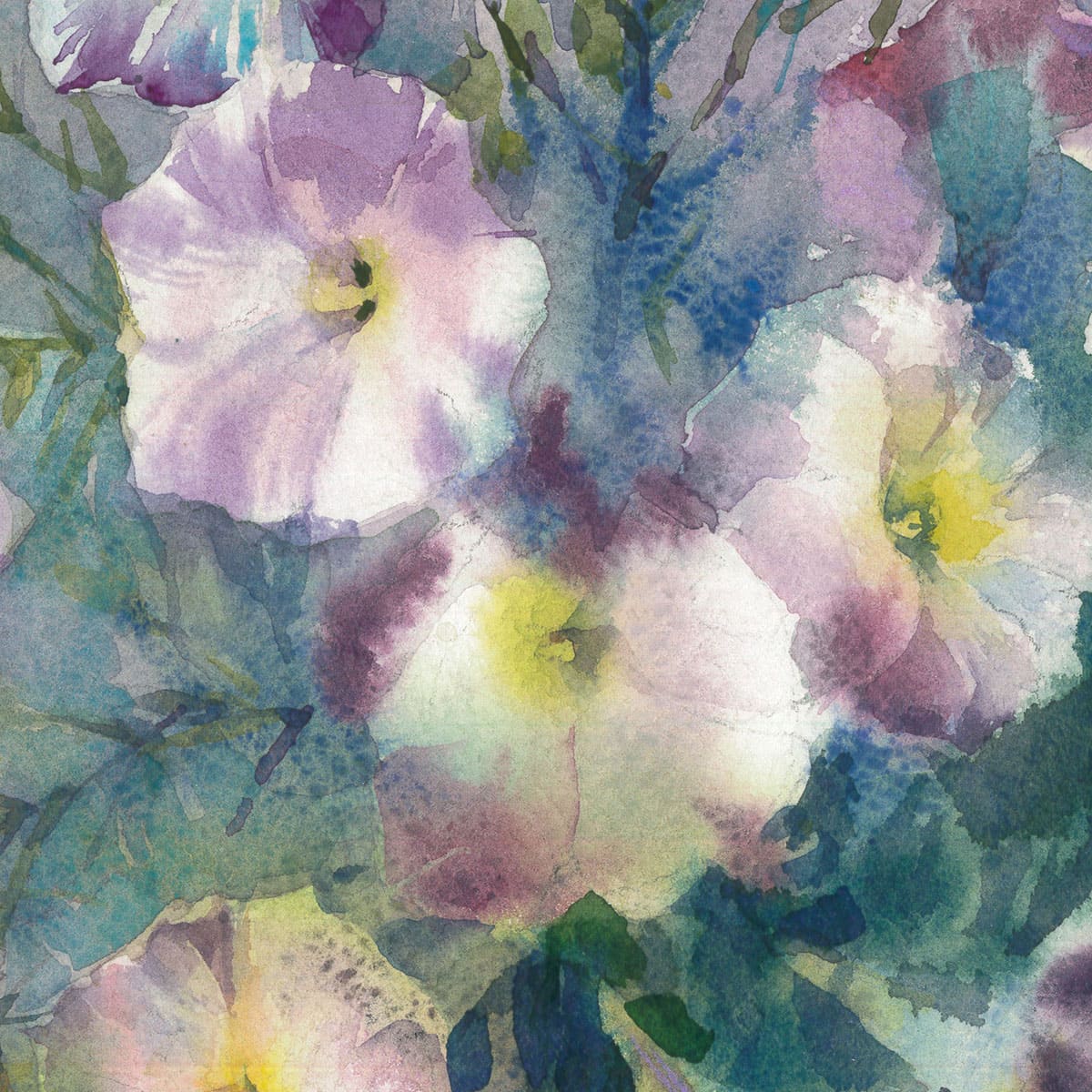This image showcases a delicate and ethereal watercolor painting of flowers, rendered in soft, pastel hues. The canvas is filled with an abstract array of colors, featuring delicate lavender, dark purple, and white petals with faded gold centers accented by small black spots. The flowers, numbering around three to four full blooms along with partial glimpses of others, stand out against a blurred, Impressionist background of pale green, blue, and purple foliage. The painting exudes a floaty, otherworldly quality, capturing a slightly unnatural but intensely beautiful bouquet. The details are diffuse and smudged, giving the impression of a fleeting, dreamy glimpse into a garden scene, with no additional elements or text present.